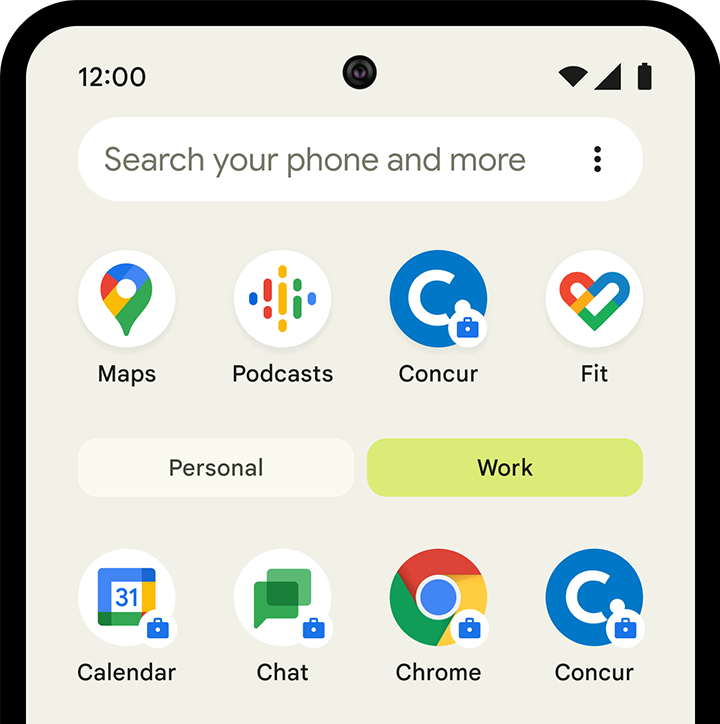This image is a partial screenshot of a smartphone home screen, specifically highlighting the sections for organizing apps into 'Personal' and 'Work' categories. The captured screen shows the top half of the phone, with the time displayed as 12:00 PM and a central camera sensor located at the top edge. Underneath the time, there is a search bar labeled "Search your phone and more."

Below the search bar, there are app icons arranged in a grid. The visible icons include Maps, Podcasts, Concur, and Fit. Below these icons, there are two tabs labeled 'Personal' and 'Work,' indicating that the user can switch between personal and work-related applications.

When the 'Work' category is selected, the icons displayed include Calendar, Chat, Chrome, and Concur. Conversely, selecting the 'Personal' category shows icons for Maps, Podcasts, and Fit. The distinction between the categories is marked with an icon resembling a briefcase, suggesting a professional setting. This icon might also imply a lock feature, although it's not entirely clear from the screenshot.

Overall, the screenshot demonstrates the convenience of toggling between personal and work modes on the smartphone, highlighting the organized separation of applications based on their intended use.